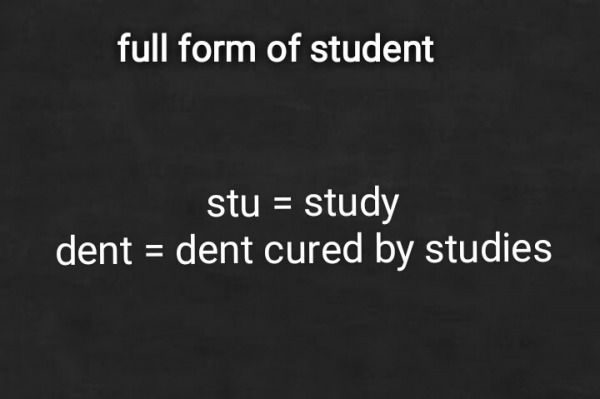This image, featuring a black background slightly faded with varying shades of black, displays text in white lowercase letters. At the top, off-center to the left, it reads "full form of student." Below, centered in the middle of the image, are two lines of text: "stu equals study" and "dent equals dent cured by studies." The overall design resembles a chalkboard with printed words, invoking an academic feel despite the text's digital appearance. The alignment creates a visual hierarchy, with the explanatory phrases forming a balanced, center-justified block, contrasting the slightly misaligned introductory phrase at the top.